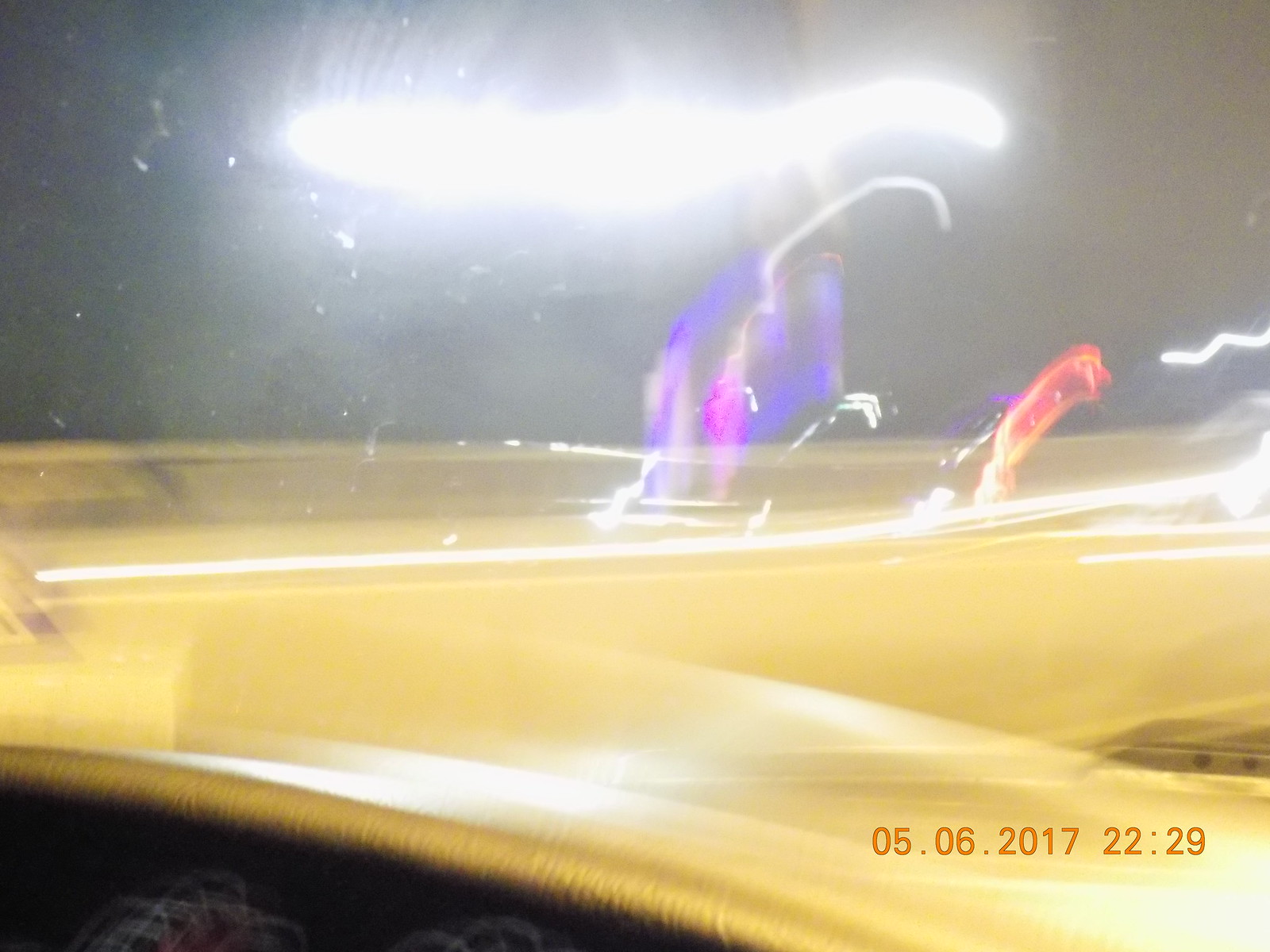The image depicts a scene captured at night, viewed through a windshield while driving swiftly down a highway or freeway. The photograph is blurry, likely due to the speed and movement of the vehicle. Central to the image is a bright, shiny yellow object, which appears illuminated by various colored lights. At the top of this object, there are glowing blue, purple, and orange lights, while a horizontal white light emanates from its center. The left side of the image features small white lines against a dark background, contributing to an impression of motion.

Below the central object, a wavy yellow-white pattern suggests the illusion of flowing liquid or a reflection. To the bottom left, a dark area is interspersed with red and white lights. On the bottom right corner, there is a date and time stamp written in brown, displaying "05-06-2017" and "22:29". The dashboard of the vehicle appears light tan, with some black illuminated elements. The combination of fast-moving reflective lights—including blue, pink, and red—across the windshield, alongside white laser-like streaks, collectively creates an illusion reminiscent of a flying saucer in the sky with beams of light emanating from it.